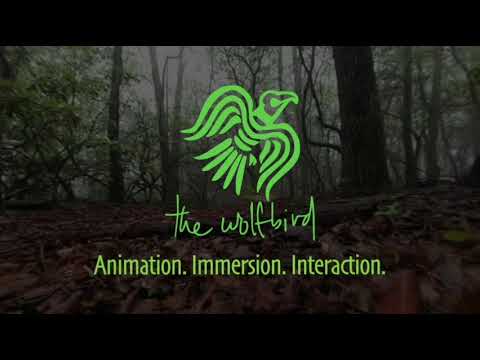The image is an advertisement displaying a forest scene with a dark and somewhat eerie ambiance, featuring trees with green leaves and brown or gray trunks, and leaves scattered on the ground. Central to the image is a bright neon green bird logo, formed out of sleek, green lines and appearing to fly vertically. Overlaid beneath the bird in elegant, cursive script is the text "The Wolf Bird" in a slightly different shade of green. Below this, in a standard font, it reads "Animation Immersion Interaction," also in green. The logo and text are centrally positioned against the forest backdrop, with a black border running along the top and bottom of the image, framing the scene.